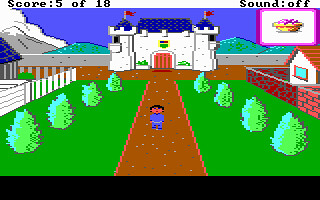This image appears to be a screenshot from an older cartoon-style video game. The interface includes a white bar at the top with black text: "score 5 of 10" on the left and "sound off" on the right. A black bar resides at the bottom of the screen. The scene depicts an outdoor courtyard with a straight brown dirt pathway flanked by green grass and light green bushes. A character with dark hair, dark skin, and dressed in all blue is walking towards the screen. On the left side, there's a building with blue roofs and grey walls, while the building on the right side features a brown roof and white walls; both are positioned in the background. The left side also has a white fence, and the right side showcases two shades of red brick fences, with the lighter shade in the front. A prominent white castle with dark blue roofs, each topped with a red flag, stands in the background. Two turrets mark its corners, and a central arched double door is visible. Behind the castle, teal-colored mountains, including one with a snow-covered peak on the far left, stretch across the horizon under a light blue sky and fluffy white clouds. Additionally, in the upper right-hand corner is a pink square with a white center featuring an image, possibly of a bowl or pie. The detailed and colorful landscape, coupled with the clear vintage interface elements, captures the nostalgic charm of early video games.